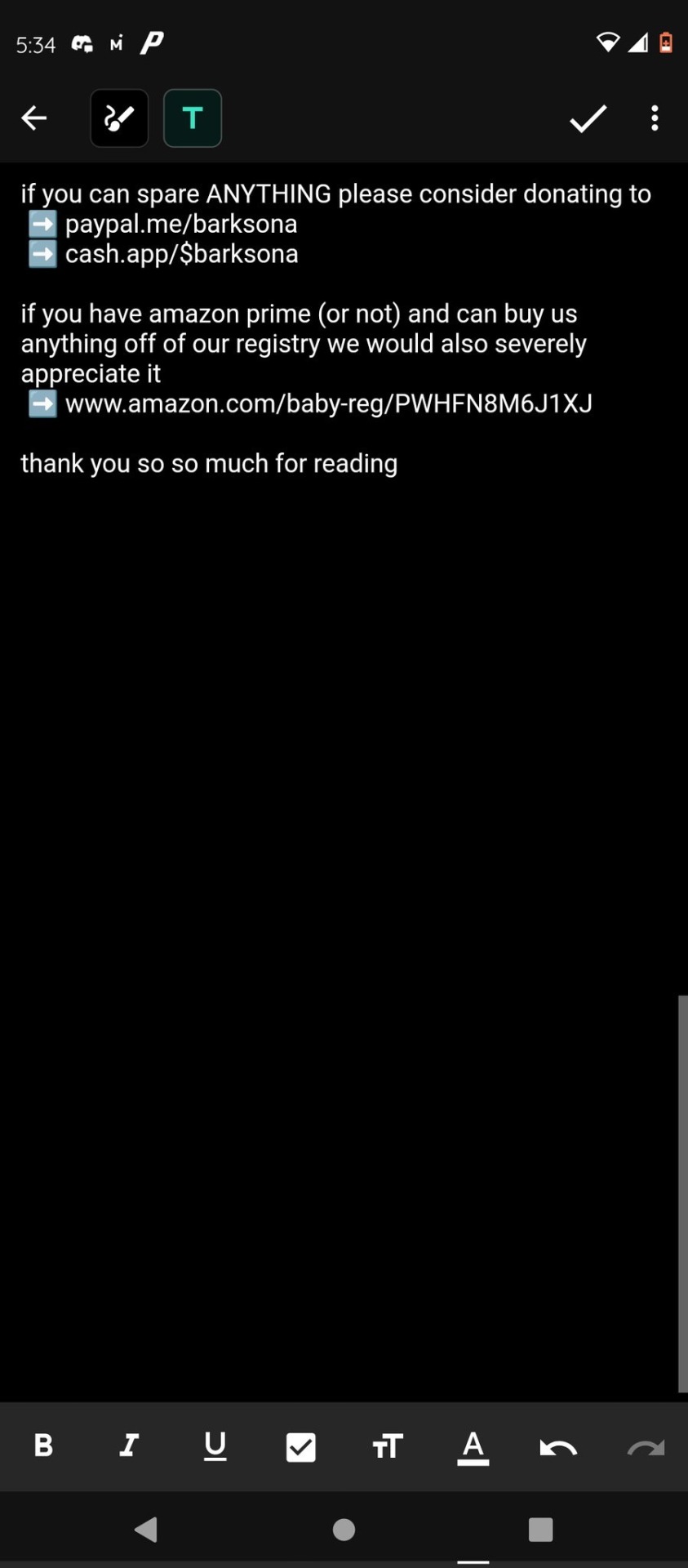This image captures a screenshot from a cell phone display. The background is entirely black, and most of the lower portion of the screen is also black. At the top, a series of white text messages can be seen. If you zoom in, the text reads: 

"If you can spare anything, please consider donating to" followed by an arrow pointing to the right, directing to the link "paypal.me.barksona". Beneath that, another arrow points to the right, leading to "cash.app/$barksona". 

Further down, there's a space before another message reads: "If you have Amazon Prime (or not) and can buy us anything off of our registry, we would also severely appreciate it." This is followed by a link to their Amazon registry, specifying "baby-reg" with a long identification number. The message ends with a "Thank you so much for reading."

At the top of the screen, the time is displayed as 5:34, though it's unclear whether it's AM or PM. There are some icons at the top, and the battery symbol, which is orange, indicates it's approximately 20% charged.